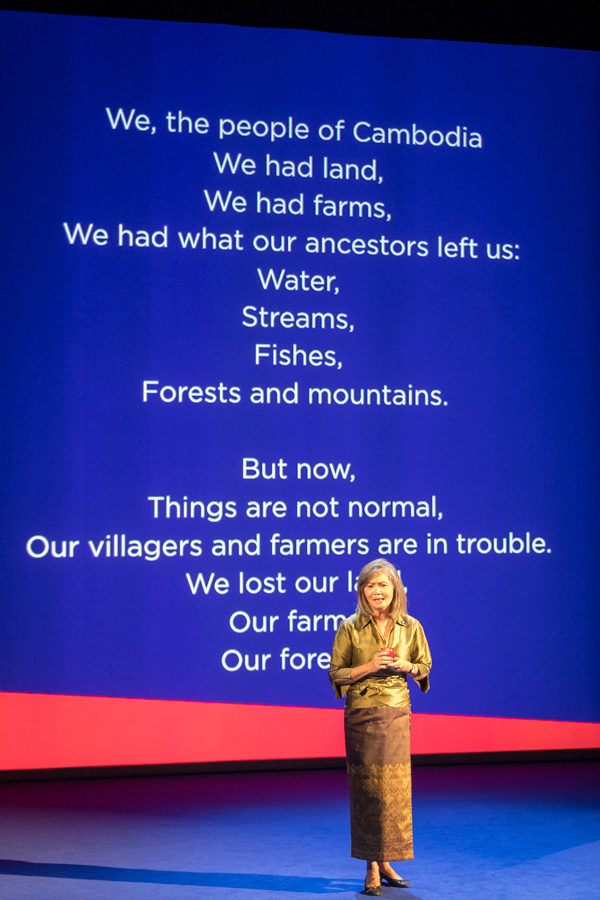In the image, an older Asian woman, likely in her 50s or 60s, stands on a stage delivering a presentation. She has long, shoulder-length brown hair and is wearing a long gold dress that extends down to her ankles, complemented by matching golden shoes. Her hands are clasped together at her chest as she looks to her right, illuminated by a spotlight. Behind her is a large blue screen with white text that reads: "We the people of Cambodia, we had land, we had farms, we had water, streams, fishes, forests, and mountains our ancestors left us. But now things are not normal. Our villagers and farmers are in trouble. We lost our land, our farmers, our ___," with the last word obscured by her figure. The screen also features a red triangle at the bottom, adding a touch of color to the predominantly blue background. The stage is otherwise bare, highlighting her presence and the urgent message displayed.